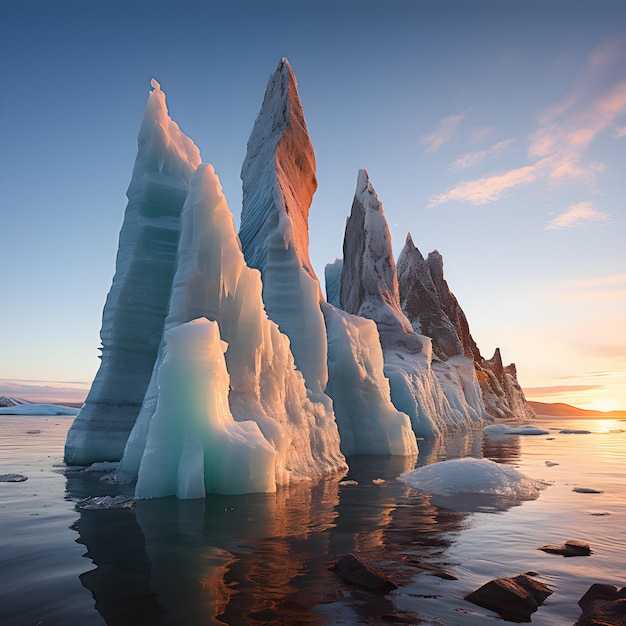This detailed photograph captures an iceberg floating in the serene ocean, its intricate, triangular ice peaks piercing through the calm, reflective water. The iceberg displays contrasting textures, with some ice structures appearing bright white and others stained with dirt. In the tranquil water, where the blue sky and minimal, wispy clouds above mirror perfectly, the deeper, concealed portions of the iceberg hint at its immense, hidden mass below the surface.

Landfall is visible in the distance, revealing a picturesque valley flanked by hills, presumably leading to a glacier or snow drift. The soft hues of the landscape contrast against the clear, blue sky, which intensifies in color towards the top. On the right side of the image, the sun has just cleared the horizon, casting a gentle, golden light across the scene, suggesting the early moments of sunrise. The combination of natural elements – the monumental ice, the placid water, and the serene sky – creates an almost surreal, computer-generated quality, despite being a true testament to nature’s artistry.